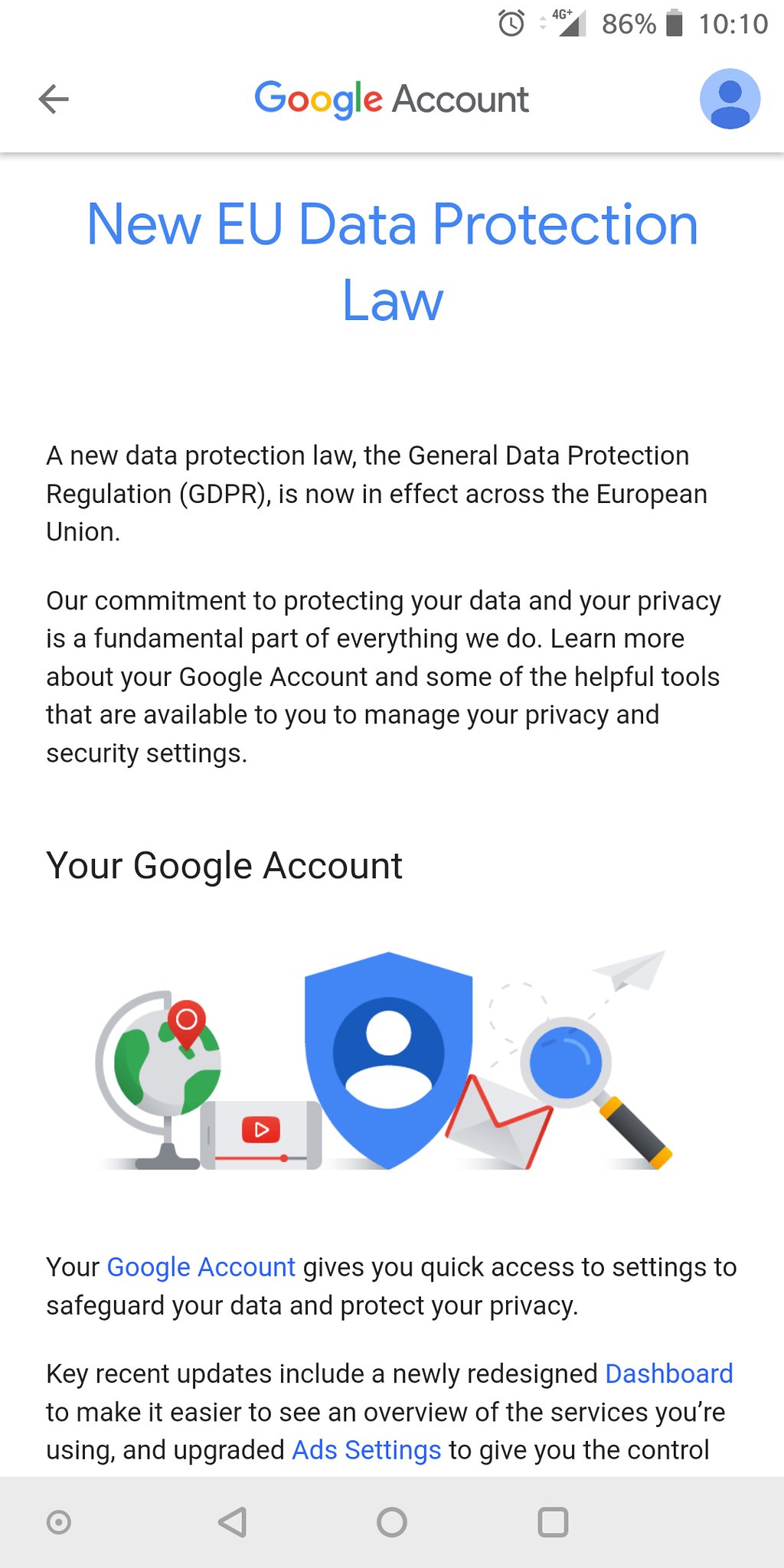The image is a screenshot of a Google account page, featuring a detailed overview of account information alongside graphical elements. 

### New EU Data Protection Law
The headline, prominently displayed in blue, introduces the primary topic. Below this, there is an extensive body of text that details the implications of this new regulation.

### Your Google Account
Beneath the initial text, a smaller black headline states "Your Google Account," leading into a section that includes several stylized graphics. 

- **Globe with a Red Teardrop Pin**: This likely represents location or global reach.
- **Rectangular Image with Triangle on a Red Background**: Possibly an icon for media or digital content.
- **Blue Shield with Person Icon**: This symbolizes user security or protection settings.
- **White Envelope with Red Border**: Suggestive of email or communication functions.
- **Magnifying Glass**: Represents search functionality.
- **Paper Airplane**: Typically associated with messages or quick actions like sending information.

### Interactive Links
The page includes several clickable links, identifiable by their blue text. Important links mentioned are: "Google Account," "Dashboard," and "Ad Settings."

### Status Bar
At the very top of the screenshot, the status bar reveals additional information:
- Time: 10:10
- Battery Level: 86%
- Connectivity: 4G

This caption offers a comprehensive and detailed description of the elements within the Google account page screenshot.